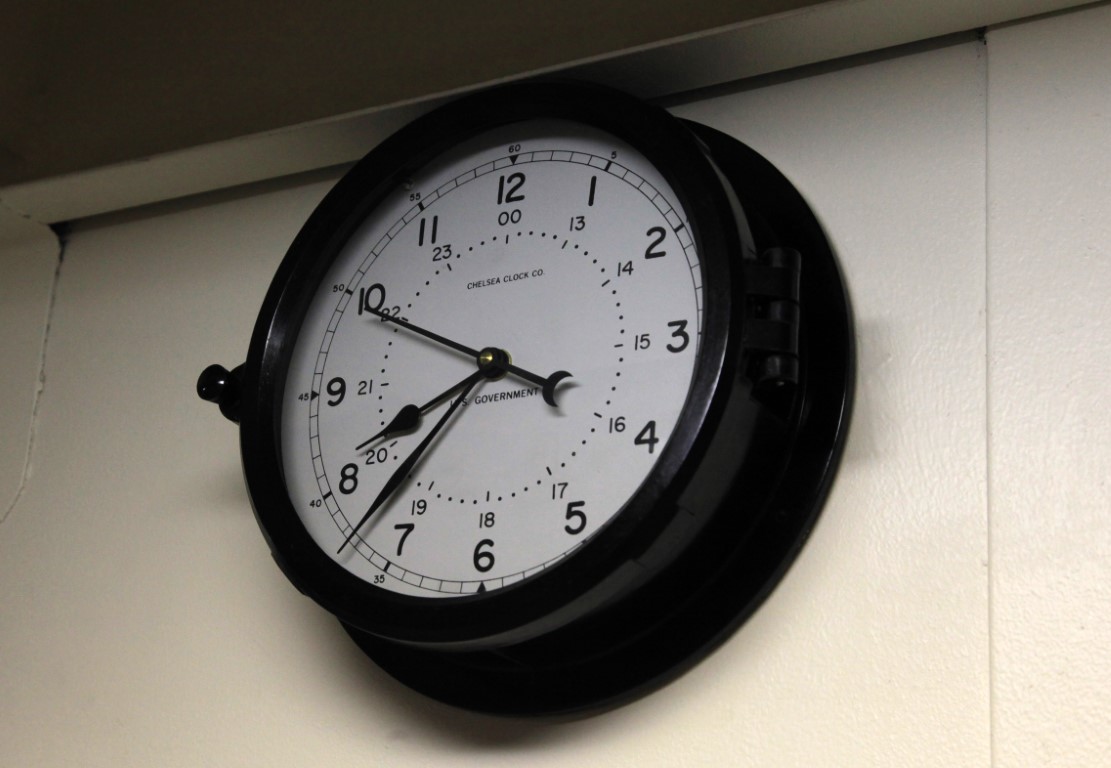The image showcases a minimalist scene dominated by a large, vintage black clock mounted on a pristine white wall. Positioned near the top edge of the wall and partially revealing the ceiling and left-hand side, the photo captures a sense of height and space. The clock, cast from steel and painted black on its outer ring, presents an aura of aged elegance. Its white clock face provides a stark contrast to the bold black numerals, hands, and dials. A notable artistic detail is the crescent moon shape of the second hand, adding a whimsical touch to the otherwise classic design. Functional elements like a hinge on the right side and a handle on the left suggest that the clock is designed for easy winding and maintenance, encapsulating both form and function in this timeless piece.